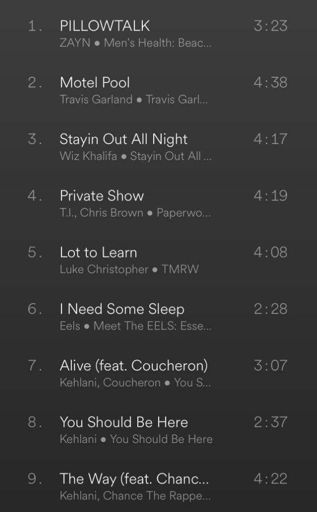This image is a screenshot of a music playlist displayed with a dark gray or black background and white text. It showcases a table format with multiple columns and nine rows, each representing a different song. The columns include the song's number, title, artist, additional descriptions, and duration. Here's a detailed breakdown of the songs featured in this playlist:

1. **"Pillow Talk" by Zayn**  
   - **Description**: Men's Health, Beach (partially visible)  
   - **Duration**: 3 minutes, 23 seconds

2. **"Motel Pool" by Travis Garland**  
   - **Duration**: 4 minutes, 38 seconds

3. **"Staying Out All Night" by Wiz Khalifa**  
   - **Duration**: 4 minutes, 17 seconds

4. **"Private Show" by T.I. featuring Chris Brown**  
   - **Duration**: 4 minutes, 19 seconds

5. **"Lot to Learn" by Luke Christopher**  
   - **Album**: TMRW  
   - **Duration**: 4 minutes, 8 seconds

6. **"I Need Some Sleep" by Eels**  
   - **Album**: Meet the Eels: Essential Eels  
   - **Duration**: 2 minutes, 28 seconds

7. **"Alive" featuring Coucheron by Kehlani**  
   - **Duration**: 3 minutes, 7 seconds

8. **"You Should Be Here" by Kehlani**  
   - **Album**: You Should Be Here  
   - **Duration**: 2 minutes, 37 seconds

9. **"The Way" featuring Chance the Rapper by Kehlani**  
   - **Duration**: 4 minutes, 22 seconds

The table is meticulously organized, presenting a clear structure for the playlist's content.